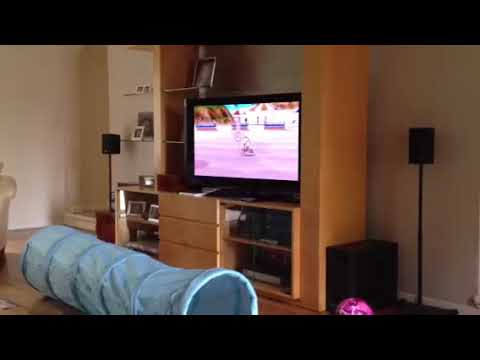This image showcases a cozy and detailed living room scene. At the center, there is a black TV mounted on a light brown wooden entertainment center, which features various open and closed storage compartments. The entertainment center houses multiple electronic devices, including what appear to be VCRs or DVDs and another black box. 

On the left side of the entertainment center, framed photos are prominently displayed on the top shelf, while the bottom shelf has white containers. In front of the entertainment center, there's a blue tunnel toy—likely for a cat or possibly a baby to crawl through. Standing tall on either side of the entertainment center are black, vertical rectangular speakers, elevated on thin poles with sturdy bases.

The TV appears to display a video game scene, showing a character racing a car in a pink mist. Adjacent to the TV on the bottom right, there's a black, vertical device resembling a PC box, accompanied by the top half of a pink soccer ball. The room features elegant hardwood floors and pristine white walls, adding to its inviting atmosphere. Only the edge of a couch is visible in the frame, suggesting additional comfort and seating in this well-equipped living space.